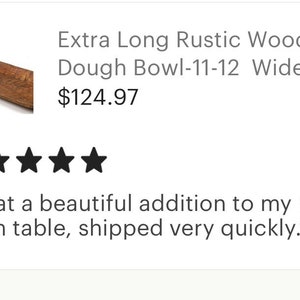The image is a square with a white background, making it difficult to see the edges clearly. At the very top, there's a light gray horizontal line stretching from left to right across the entire width. 

On the left side of the image, there is a square object that looks like a piece of wood, possibly a cutting board, oriented at an angle around 7:30. The wood has a medium brown color.

To the right of the wooden square, there's gray text in a large font. The first line reads "extra long rustic woo" (with the last letter 'D' missing, likely implying "wood"). The second line of text says "doble dash 11-12 wide", with the 'E' in "wide" partially cut off.

Directly below this text, the price "$124.97" is displayed. Further down, below the price, there are star ratings, where four stars are shown but the last one on the left is partially cut off. Beneath the star ratings, there is smaller text that states, "add a beautiful addition to my", and the line below says "table, shipped very quickly."